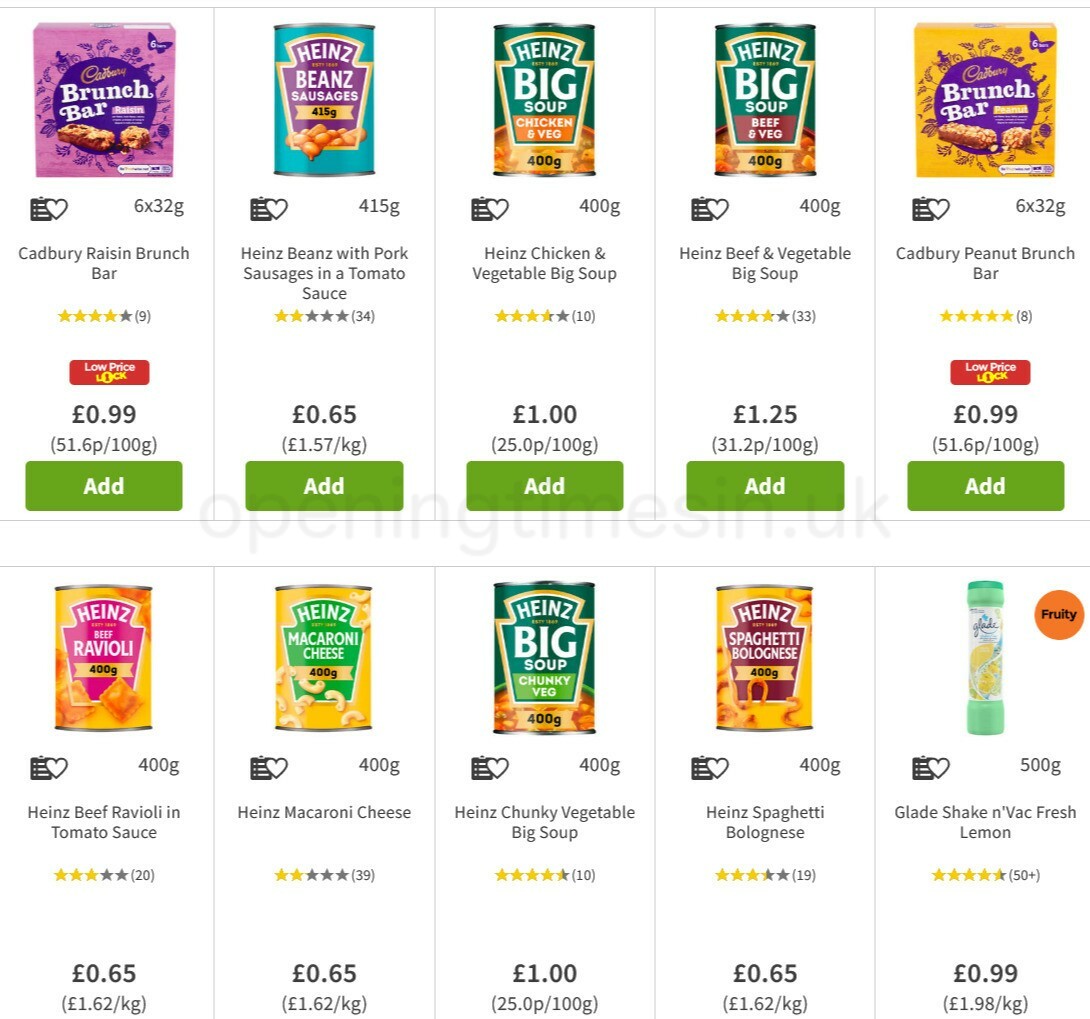**Description:**

Screenshot of an online shopping page displaying a watermark across the center that reads "openingtimesin.uk". The layout features two rows of products, each containing five distinct items. 

**Top Row:**

1. **Product 1:** A pink box with a purple logo labeled "Brunch Bar".
2. **Product 2:** A blue can with a purple label, identified as "Heinz Bean Sausages".
3. **Product 3:** A green can marked "Heinz Big Soup" (center item).
4. **Product 4:** Another green can labeled "Heinz Big Soup".
5. **Product 5:** A yellow box with a purple label, also identified as a "Cadbury Brunch Bar".

Each product includes a small photo, the name of the product, customer reviews, and the price. The items in the top row feature a green "Add" button at the bottom for quick purchase.